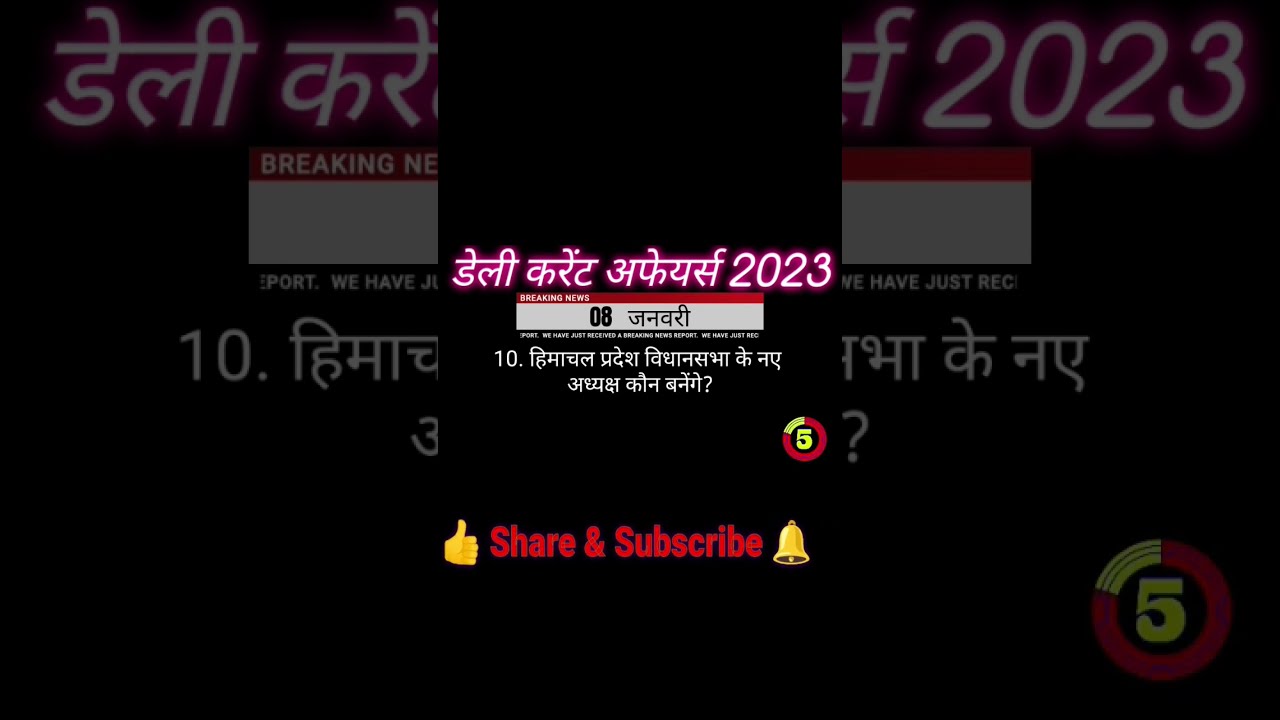The image is a detailed screenshot of a YouTube video in an Indian language, appearing to be of breaking news from 2023. The visually striking centerpiece is the neon lavender font, glowing against a black background, with text in an Indian script. Below it, a gray rectangle prominently displays the number 08 in black. Just above this, sits the number 10 in white, surrounded by additional Indian writing. On the right side, a circular logo is divided by thin black lines into sections that are predominantly red with a small yellow portion, and it features a cartoonish yellow number 5 in the center. At the bottom, red text commands viewers to "share and subscribe," accompanied by a yellow thumbs-up emoji on the left and a yellow bell emoji on the right. All elements appear upright, suggesting the screenshot was taken on a mobile phone.